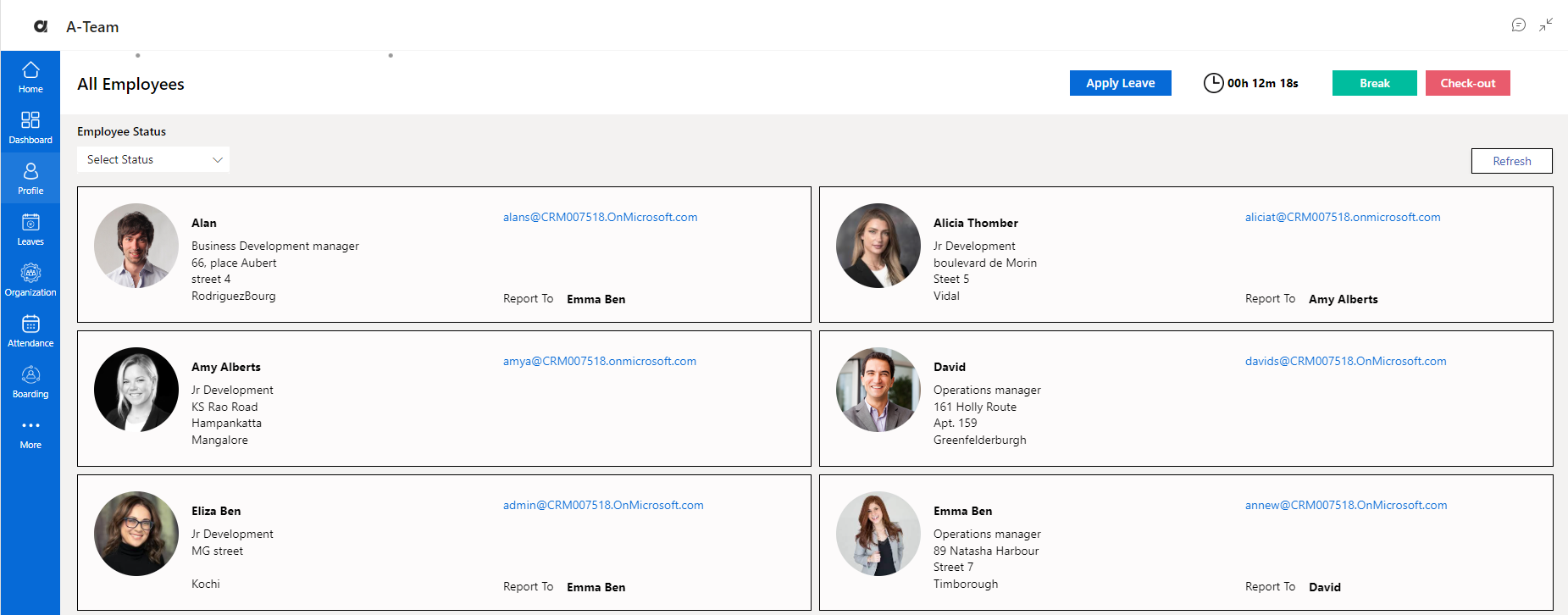In this image, we see a detailed page of an application or website with the header labeled "A-Team" in the top-left corner. The header includes the black "A" logo. On the top-right corner, there are several buttons, including a prominent blue button labeled "Apply Leave" and a countdown timer displaying 00 hours, 12 minutes, and 18 seconds. Additionally, there are two action buttons: a green "Break" button and a red "Check Out" button.

On the left side of the page, there's a menu icon with a blue background. The menu options include Home, Dashboard, Profile, Leaves, Organization, Attendance, Boarding, and a "More" button. The Profile menu item is currently selected.

The main content area under the Profile section features a light grey background with a text header reading "All Employees" and a dropdown menu labeled "Employer Status" for filtering employee statuses. To the right side of this section, there is a white refresh button.

The page lists six employee profiles:

1. **Alan** - Business Development Manager, located at 66 Place Albert Street 4, Rotary Cross Park. The profile also contains his email address.
2. **Ami Albert** - Junior Developer.
3. **Eliza Penn** - Junior Developer.
4. **Alicia Tomba** - Junior Developer.
5. **David** - Operations Manager.
6. **Emma Penn** - Operations Manager.

All the employees listed use an email address ending in "@microsoft.com".